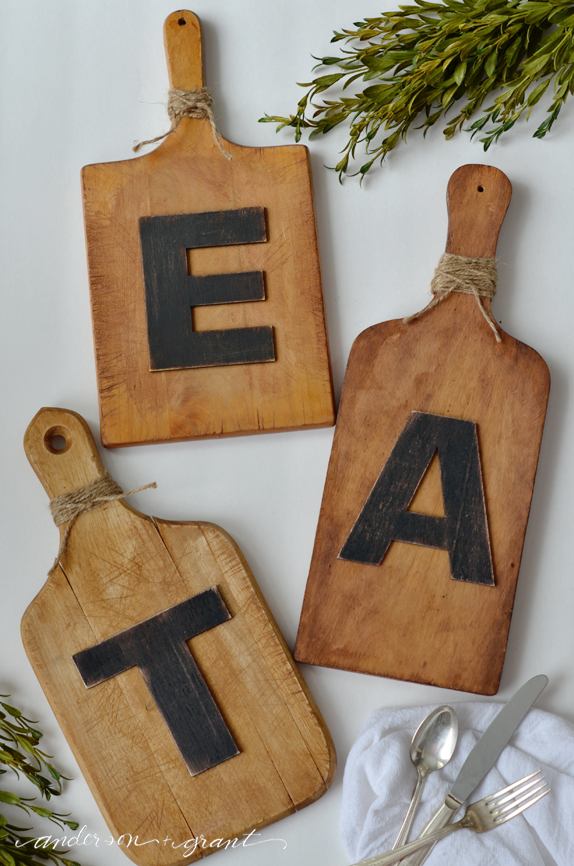This image showcases a trio of rustic cutting boards, each adorned with a bold black letter, together spelling out the word "EAT." The cutting boards vary in shapes and wood shades; one is square-shaped with an 'E' and is more straight-edged, another is lighter with a rounded top and a 'T', and the third is longer, darker, and curved at the top, featuring an 'A'. Each board has a rope tied around its neck, enhancing the rustic charm. They are laid flat on a white tablecloth, with sprigs of greenery in the upper right and lower left corners, alongside a set of silver utensils (spoon, knife, and fork) resting on a white dish towel at the bottom right. A photographer's watermark reading "Anderson Grant" in white cursive is visible in the lower left corner.